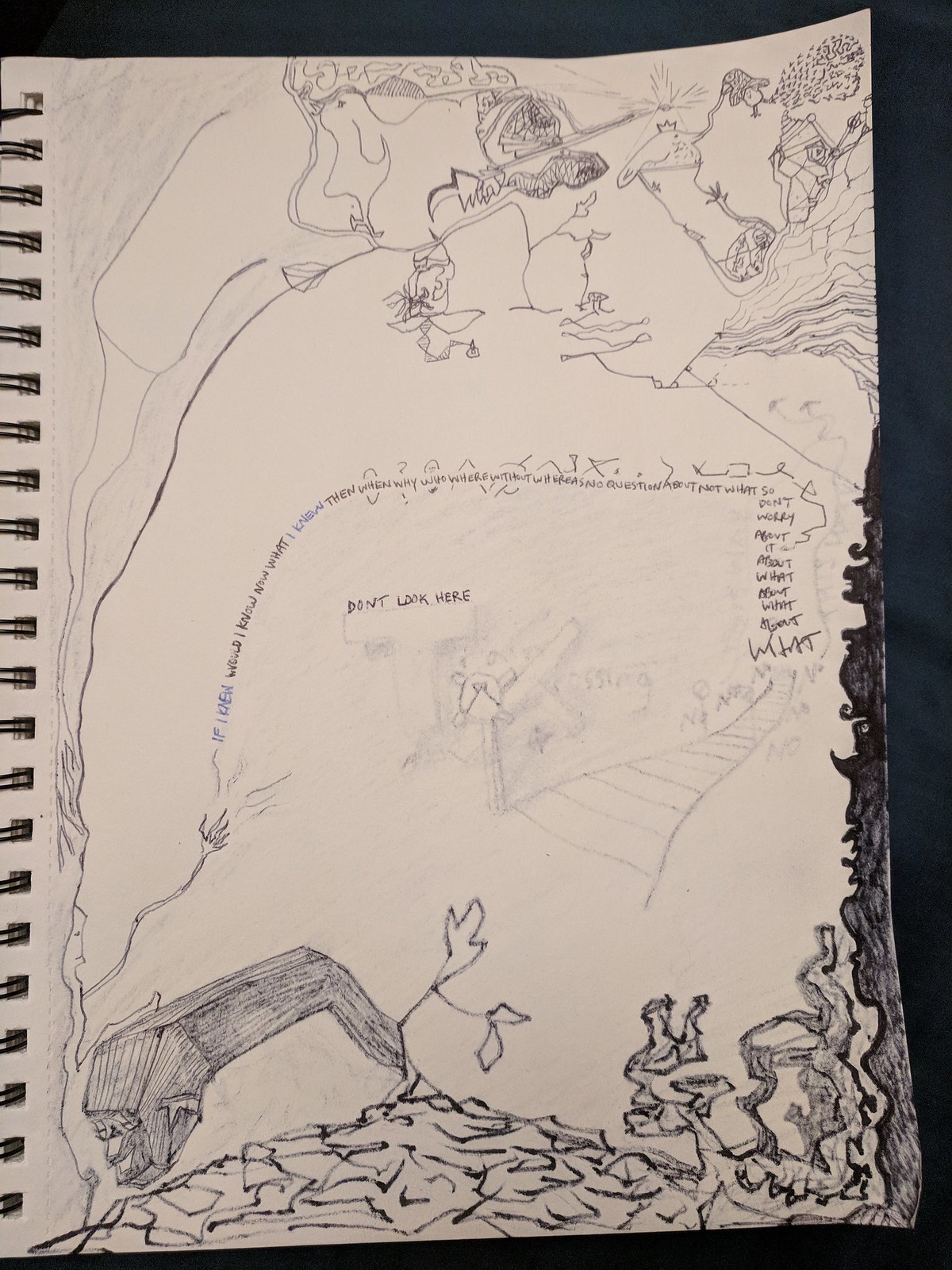The photograph showcases a well-used spiral-bound notebook resting on a dark fabric background, likely a deep blue or black, with visible ripples indicating it's some form of cloth. The notebook page is filled with handwritten text, the most prominent phrases being "don't look here" and a sequence of partially decipherable words and phrases such as "if, when, something, something, no, no, no." The text is generally illegible due to its small size and dense arrangement. Additionally, the page is adorned with various intricate drawings: a peculiar rock-like character occupies the bottom-right corner, vines extend along the right edge, and what appears to be a small tree emerges from the top-right of the page. The upper section of the page features a collection of different characters, and a pencil sketch of a road is also visible. The overall style is a mix of pen and pencil illustrations and handwritten notes, capturing a moment of creativity and thought in a single notebook page.